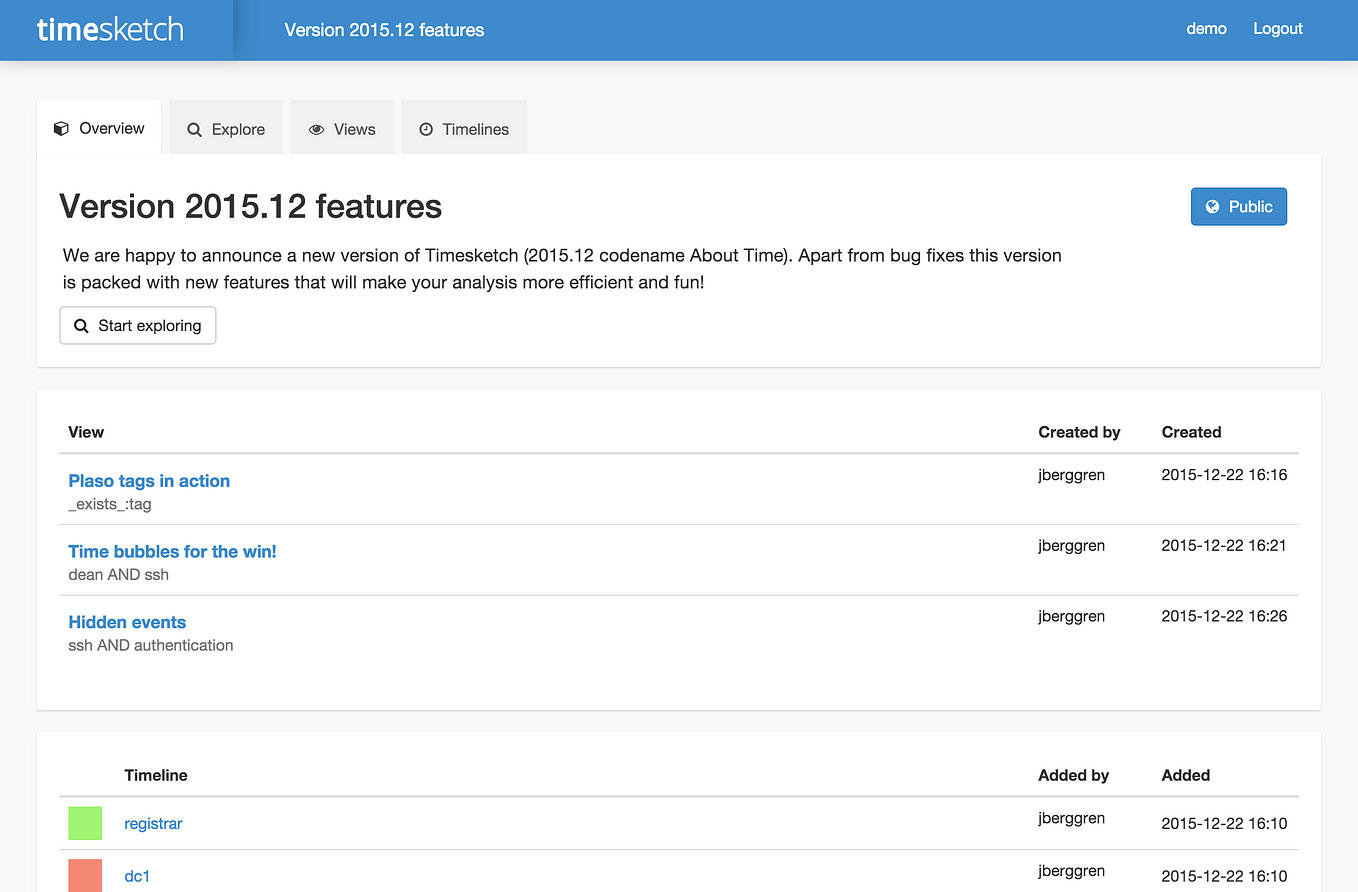The image displays the main page of the TimeSketch program, specifically showcasing the version 2015.12 features. At the top center of the screen, the header reads, "TimeSketch version 2015.12 Features." In the top right corner, there are options labeled "Demo" and "Logout."

Below these options, a navigation menu contains four tabs: Overview, Explore, View, and Timelines. The Overview tab is currently selected and provides the following information:

"Version 2015.12 features. We are happy to announce a new version of TimeSketch. Apart from bug fixes, this version is packed with new features that will make your analysis more efficient and fun."

To the right of this text, a blue button indicates that the status is public. Below the main text, there is an option to "Start Exploring."

Three different timeline entries are listed under current options to view:

- "Plazo Tags in Action," created on 2015.12.12 at 16:16.
- "Time Bubbles for the Win," created on 2015.12.12 at 16:21.
- "Hidden Events," created on 2015.12.12 at 16:26.

At the very bottom of the page, within the timeline tab section, there are two entries:

- "Registra," added by user on 2015.12.12 at 16:10.
- "DC1," added by user on 2015.12.12 at 16:10.